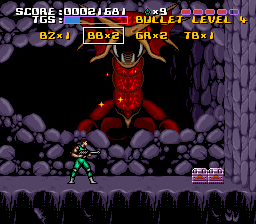A vibrant, colorful image captures a scene from an unspecified video game, likely from a console or mobile platform. The image is square and compact, with several lines of unreadable text in white, pink, and yellow at the top, probably indicating game levels or instructions. The primary setting is a cave-like area constructed from grey stones, with a stark black background that intensifies the atmosphere. Dominating the center of this cave is a vivid red monster or dragon, mouth agape, revealing formidable teeth. Below this creature, a small figure clad in green stands resolutely on a stone ledge, facing the scene. The ledge extends into a darker lower section of the image. On the right-hand side of the ledge, two tiny squares, red on the bottom and white on the top, likely serve as logos or markers, though too diminutive to decipher. The entire scene suggests a moment of tension or impending confrontation within the game.